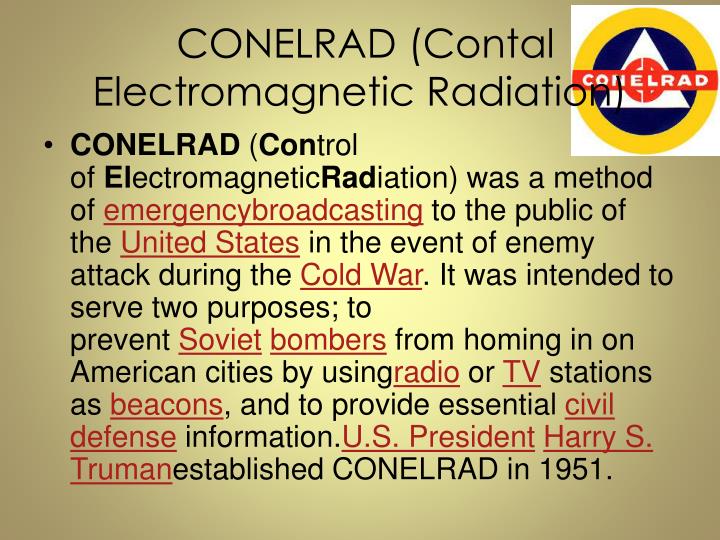The image features a background that is light tan, darkening towards the edges, with black text that prominently reads "CONELRAD (Control of Electromagnetic Radiation)." In the top right corner, there's a distinctive logo within a white box. The logo comprises a yellow circle containing a blue circle, which further encases a white triangle with a red dot at its center. Horizontally across this emblematic design is a red bar with the text "CONELRAD" in white. Below the main title, additional black text elaborates: "CONELRAD (Control of Electromagnetic Radiation) was a method of emergency broadcasting to the public of the United States in the event of enemy attack during the Cold War." Key terms such as "emergency broadcasting," "United States," "Cold War," "Soviet bombers," "radio," "TV," "essential civil defense," and "Harry S. Truman" are highlighted in red and underlined. The description specifies that CONELRAD was implemented to prevent Soviet bombers from using American radio or TV stations as navigational beacons and to provide crucial civil defense information. It was established by U.S. President Harry S. Truman in 1951.